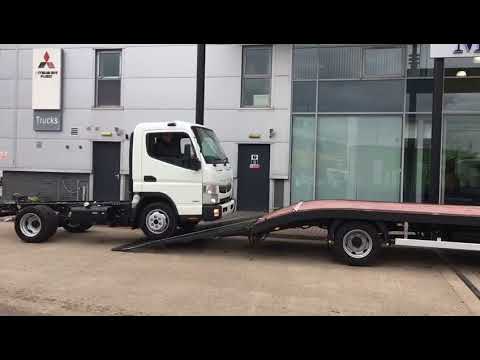In the image, a white truck with a flat front and a black truck bed is seen driving halfway up a black ramp onto the back of a larger flatbed truck, which has a light brown bed. The ramp extends from the larger truck, which is positioned towards the right side of the image, while the white truck on the ramp extends off to the left. The scene is set in what appears to be a parking lot with brown pavement in front of a gray two-story building. This building, which has numerous glass windows and black doors on its right side, serves as a notable backdrop. An additional building is visible to the left with a prominent sign that reads "trucks" in white text on a gray background, accompanied by a company logo above it. Both buildings have large glass windows with blinds or curtains partially concealing the interiors. The context suggests a car dealership or a service area where vehicles are being loaded, depending on the interpretation of the scene.